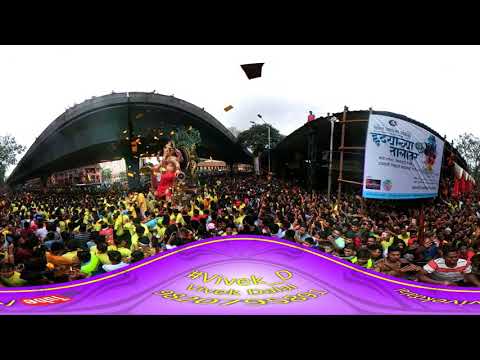The image is a panoramic shot of an outdoor concert, capturing a tightly packed crowd of hundreds of people with dark hair, creating a sea of indistinguishable faces. The photo, possibly taken with a 360-degree camera, shows a vast audience enclosed by large, curvy, stadium-like walls that emphasize the open-air setting. On the left side appears a group of people wearing yellow facing what seems to be a stage or an arched structure, while on the right side stands a long, curved wall adorned with a white banner featuring non-English writing. Along the bottom of the image, a warped purple banner with yellow writing prominently displays the hashtag "VIVEK_D" and a faint trace of a YouTube logo. The sky above is white, completing the panoramic vista of this vibrant, bustling concert scene.